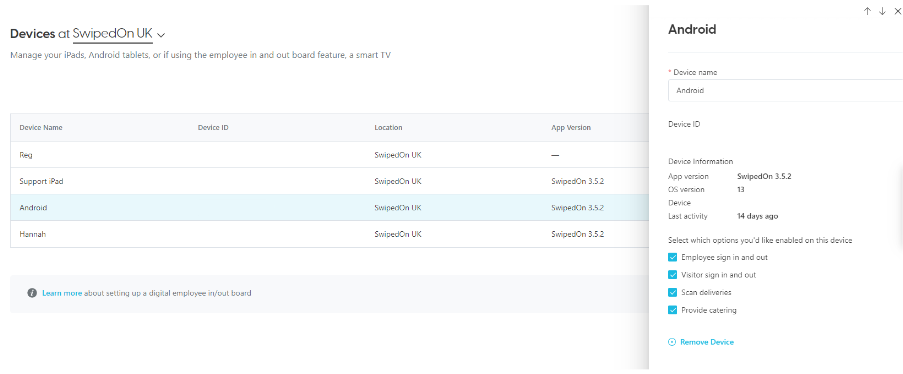**Detailed Caption:**

The image depicts a comprehensive network management tool interface designed for Bluetooth devices in an office setting. The device list features various categories, including device names, device IDs, locations, and app versions. 

The first entry, labeled "reg," does not have a specified device ID and features an app version indicated with a dash, suggesting it is inactive or unregistered. The "Support iPad" entry, also swiped in the UK, is running app version 3.5.2, highlighted in blue. A similar entry mentions an Android device at the same location, also using app version 3.5.2. Another entry for a device named "Hannah" shows it too is swiped on version 3.5.2, consistent with the others.

At the bottom, there are instructions for setting up the digital employee in-and-out port feature. On the right side of the interface, more specific details are highlighted, such as an Android device named "Android," complete with its device ID, device information, and running app version 3.5.2 on OS version 13. The device is identified as model i6v14.

The interface provides options to enable the device, sign in and out, manage visitor sign in and out, scan deliveries, and provide catering, all of which are currently checked. There's also an option to remove the device from the network, indicating the tool's functionality for managing various office Bluetooth devices efficiently.